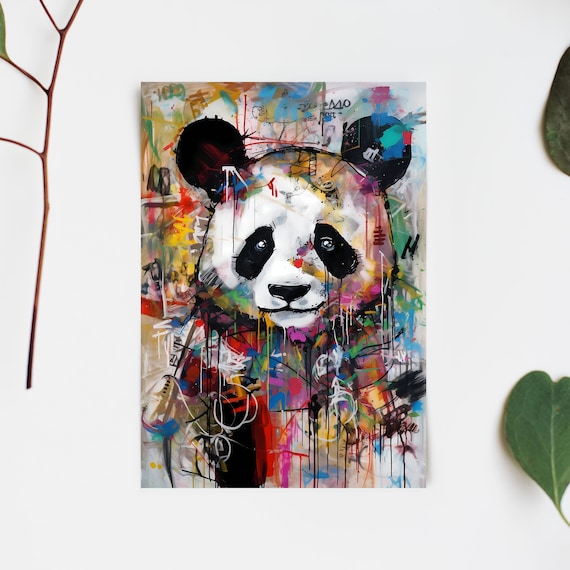This image features a striking, somewhat abstract painting of a panda bear, displayed on a rectangular canvas placed on an all-white surface. The panda's face is distinctly detailed with characteristic white fur and black markings around the eyes, ears, nose, and mouth. Surrounding the panda's face, the artwork bursts into a vibrant array of dripping paint splatters in assorted colors, including red, yellow, orange, blue, black, purple, and green, resembling a complete rainbow spectrum.

On the left side of the image, there is a skinny reddish-brown twig with a green leaf partially cut out of the frame. On the right side, towards the top, the image features another green leaf partially cut out, and at the bottom right, a third green heart-shaped leaf facing the opposite direction also partially cut out.

Additionally, the painting has some indistinct black text around it, which appears to include letters forming the start of a word, 'S-O', and what looks like a partially visible letter 'M'. The overall scene combines the striking visual of the panda with an eclectic mix of colors and natural elements, creating a dynamic and vibrant composition.